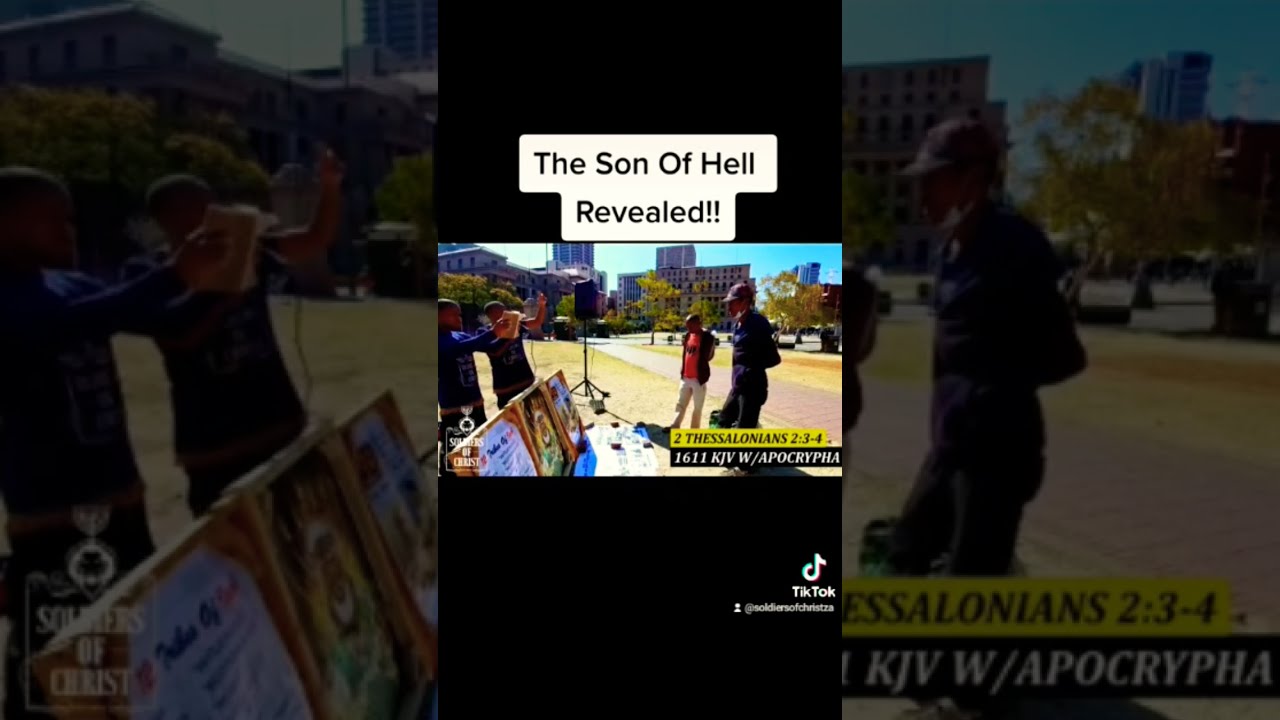The image, captured vertically on a phone, appears in the center of a widescreen format with large black bars on the top and bottom, giving it a dim and grayed-out appearance. The scene is set on a street in a town or city, featuring a sidewalk bordered by a grassy area. Four people, identified as black males, are positioned in the image: two on the left are holding up their hands and possibly speaking into a large black speaker mounted on a stand, while the two on the right are either listening or watching. Behind them are city buildings and trees, suggesting an urban environment. Notably, there are posters on the ground near the speakers, with one prominently displaying text in light green background with black lettering that includes excerpt "2 Thessalonians 2:3-4" and "1611," although the details are somewhat hard to read. At the top of the image, there is a white highlighted text stating "The Son of Hell Revealed!!".